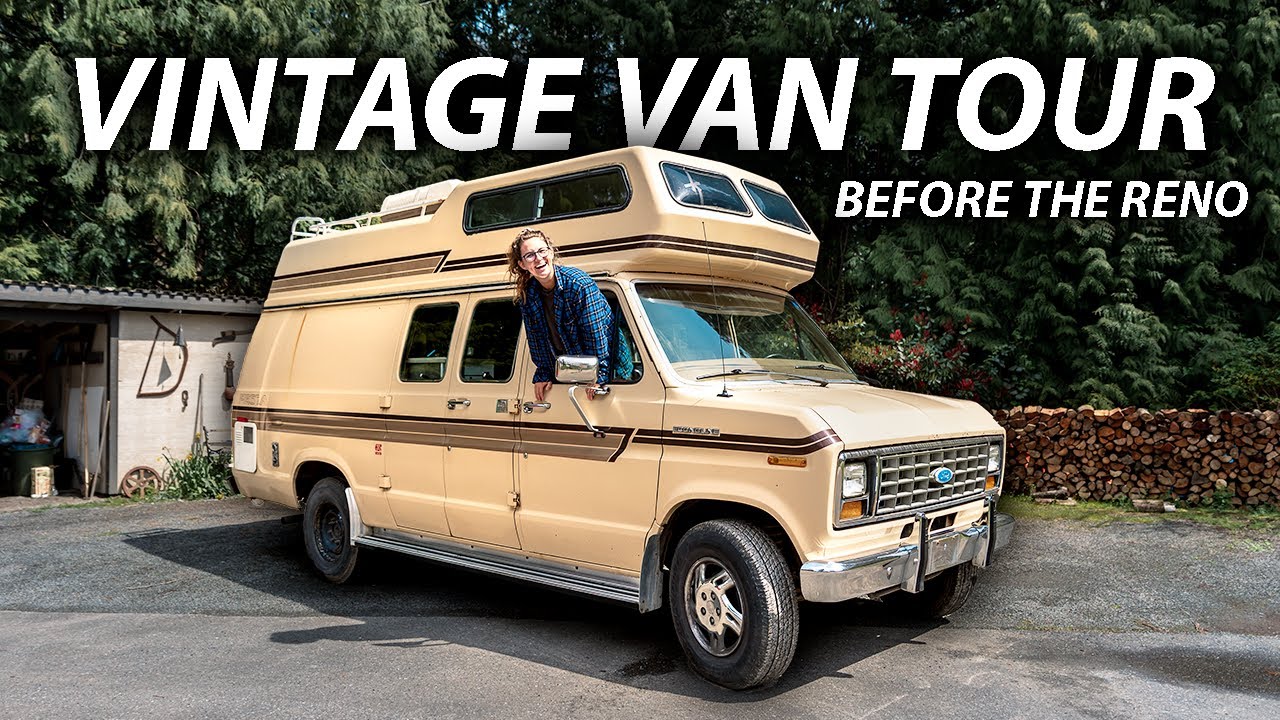In this horizontal-rectangular photograph, an old beige touring van, adorned with racing stripes and a closed luggage rack, takes center stage, parked in a driveway. Above this nostalgic vehicle, large white letters announce, "Vintage Van Tour," while smaller white text on the right reads, "Before the Reno." A woman, smiling and looking forward, leans out of the passenger window with her hands on the door, visible from her head to her waist. The van, from the 1980s, is notable for its boxy shape and vanilla tone, complemented by black and gray stripes running along its sides. Inside the van, there is a bed, and the top windows are tinted. The vehicle rests on gray and black concrete, casting a shadow beneath, and features black tires with black and silver rims, along with a blue and silver Ford emblem on the front. The background includes green trees, a white garage with a black roof, a pile of brown logs, and patches of green grass growing on the side of the driveway, all under a blue sky.